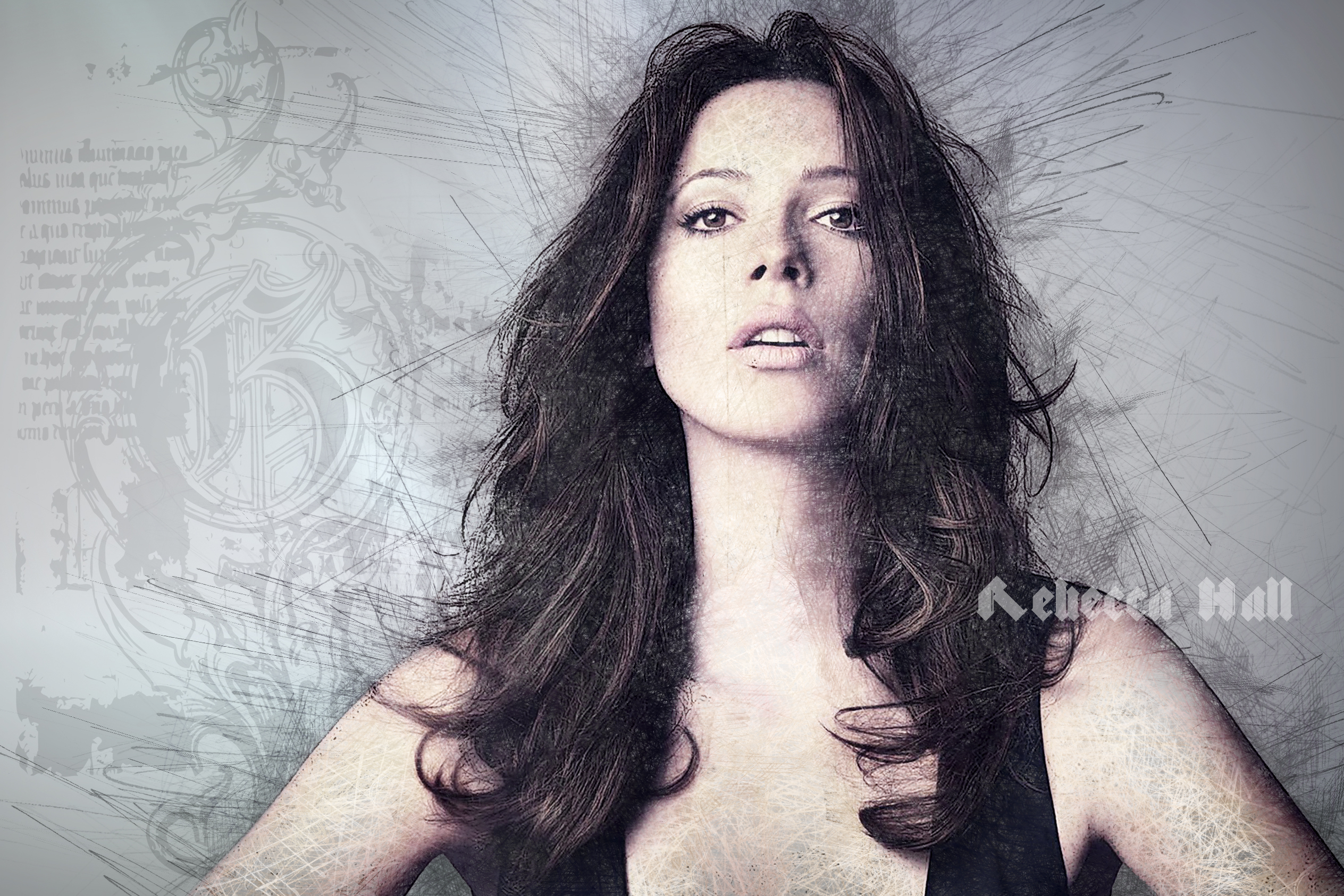This is a digitally edited color photograph of a white woman with a stylized artistic filter that gives the appearance of a chalk, charcoal, or colored pencil illustration. The woman, identified as Rebecca Hall by white text in an old-style Gothic font over her right shoulder, has pale skin, brown eyes, and long, flowing dark brown or black hair. She is wearing a sleeveless black tank top and has her head slightly tilted back with her mouth partially open, giving a poised yet candid expression. The background is a light gray adorned with barely discernible dark gray text and script that may resemble old English letters or a foreign language. Additionally, there are intricate gray line illustrations behind her head, and the left side of the image features an elaborate, indiscernible letter reminiscent of a medieval manuscript, along with lines of black text that are out of focus and unreadable.